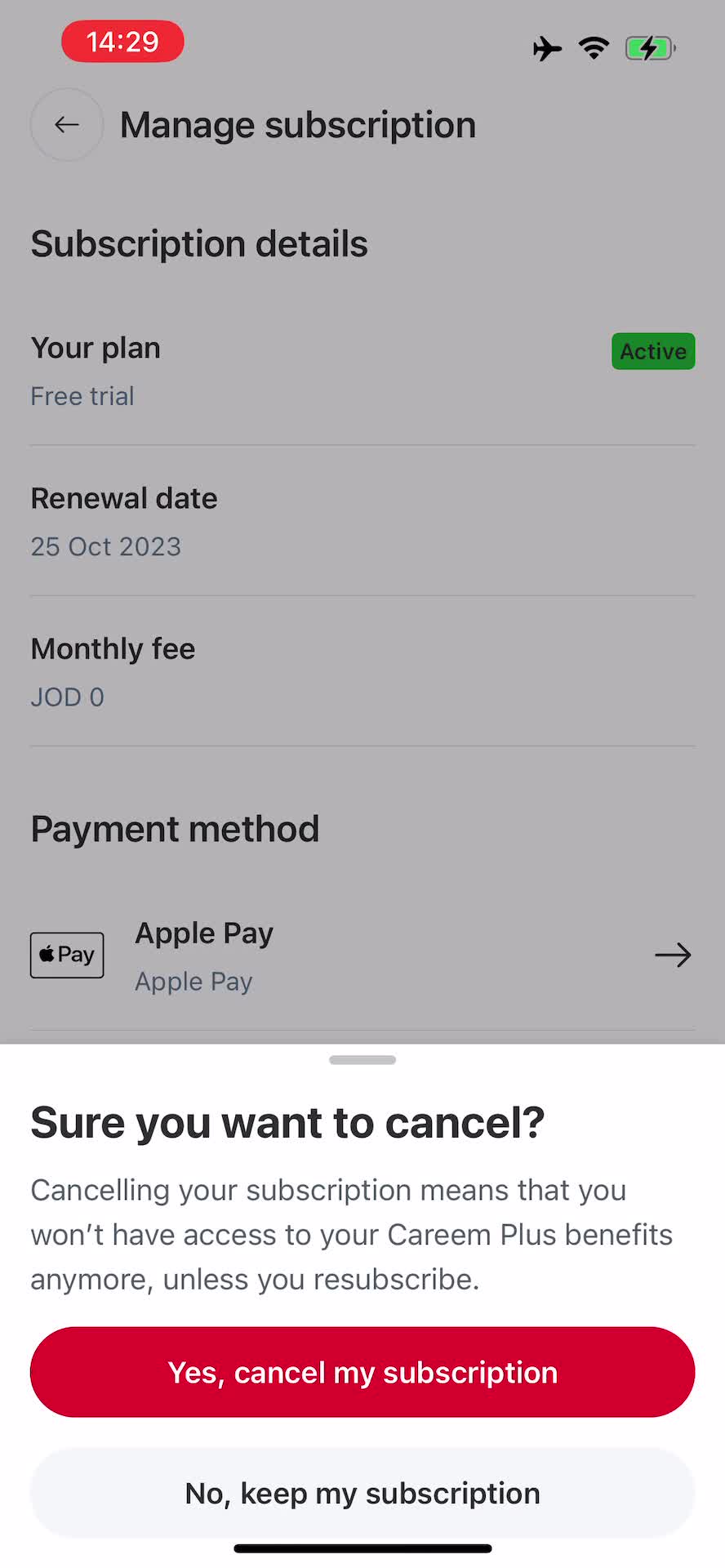This is a screen capture from a cell phone displaying a subscription management screen. The image is vertically oriented. In the upper left-hand corner, the cell phone time is visible alongside indicators for airplane mode, Wi-Fi signal strength, and a charging battery. The main heading at the top of the screen reads "Manage Subscription" in bold black letters.

Below this, there is a section titled "Subscription Details." Under "Your Plan," the screen indicates that the user is on a "Free Trial," with a solid-filled green rectangular box to the right containing the word "Active" in black letters. The "Renewal Date" is listed as 25 October 2023, and the "Monthly Fee" is denoted as "G-O-D 0." 

The next section displays the "Payment Method" as Apple Pay. There is a prompt asking, "Are you sure you want to cancel?" in bold black letters followed by a warning message in gray letters: "Canceling your subscription means you won't have access to your CREAM Plus benefits anymore unless you resubscribe."

Finally, there are two highlighted options for the user to proceed: a solid red oval button with white letters reading "Yes, Cancel My Subscription," and a light gray oval button reading "No, Keep My Subscription."